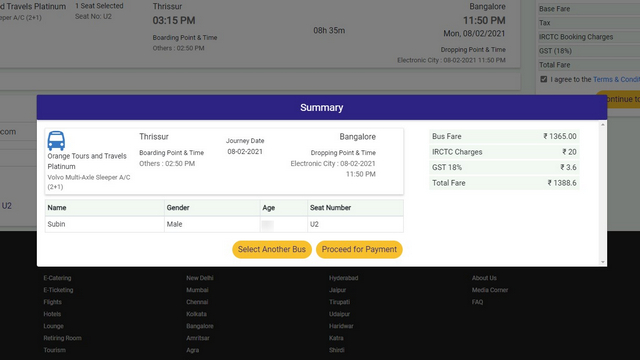The image showcases a travel website, prominently displaying booking details for a bus trip. The background features a schedule with numerous timestamps, indicating departure and arrival times. Specifically, the bus is departing from Thrissur at 3:15 PM and arriving in Bangalore at 11:50 PM. To the right, there is an order summary screen detailing the pricing. A pop-up summary reveals "Orange Tours" and a designation of "Platinum." It further specifies the route from Thrissur to Bangalore, with a bus fare of 1,365 rupees, additional charges of 20 rupees, and an 18% GST. The total cost of the trip sums up to 1,388.6 rupees.